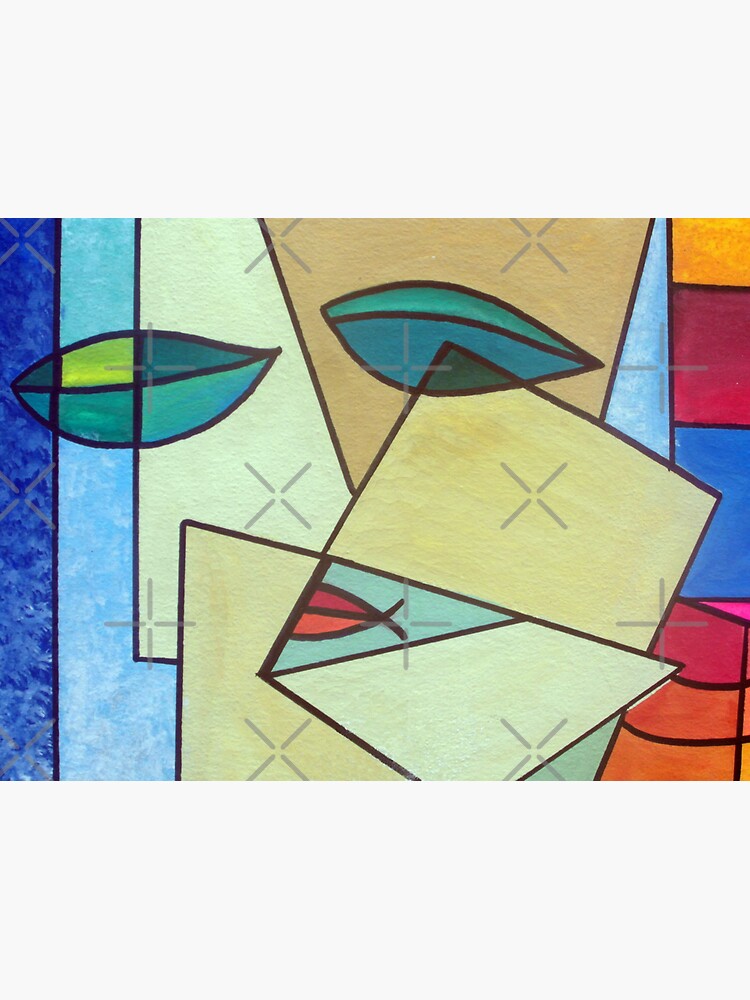This image is a vibrant, abstract art deco piece, presented in a square format. While the initial glance reveals no border, a closer inspection shows a light gray border at the top and bottom. The artwork, likely created in ink, displays a myriad of colors including light blue, black, teal, cream, red, orange, dark blue, green, tan, and yellow. The composition is marked by overlapping geometric shapes that come together to subtly hint at a face, with elements that resemble eyes formed by leaf-like shapes and lips at the center. This digital art exudes a broken-up Picasso vibe, with its colorful and dynamic arrangement, and includes digitally added X's across the image to prevent unauthorized copying.